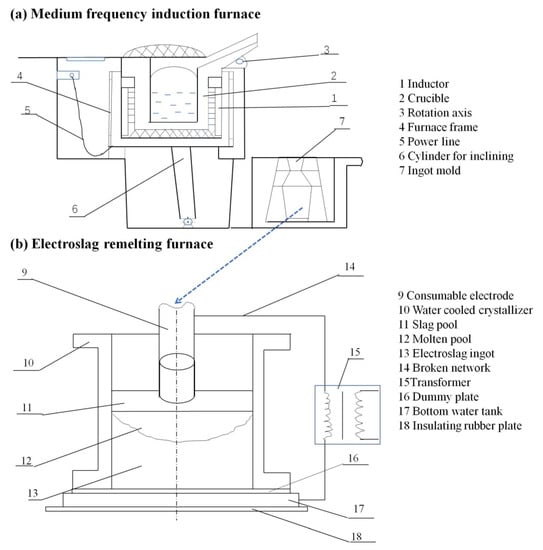This black-and-white infographic illustrates two types of furnaces with detailed diagrams and labeled parts. The top section is titled "A. Medium Frequency Induction Furnace" and features a sketch with numbered lines pointing to various components: 1. Inductor, 2. Crucible, 3. Rotation Axis, 4. Furnace Frame, 5. Power Line, 6. Cylinder for Inclining, and 7. Ingot Mold, all listed on the right side of the diagram. Below it, "B. Electro-Slag Remelting Furnace" is depicted with a sketch identifying its parts numbered from 9 to 18, which include: 9. Consumable Electrode, 10. Water-Cooled Crystallizer, 11. Slag Pool, 12. Molten Pool, 13. Electro-Slag Ingot, 14. Broken Network, 15. Transformer, 16. Dummy Plate, 17. Bottom Water Tank, and 18. Insulating Rubber Plate. These components are also listed on the right side of their respective diagram, providing a comprehensive visual guide to the structure and function of each furnace.